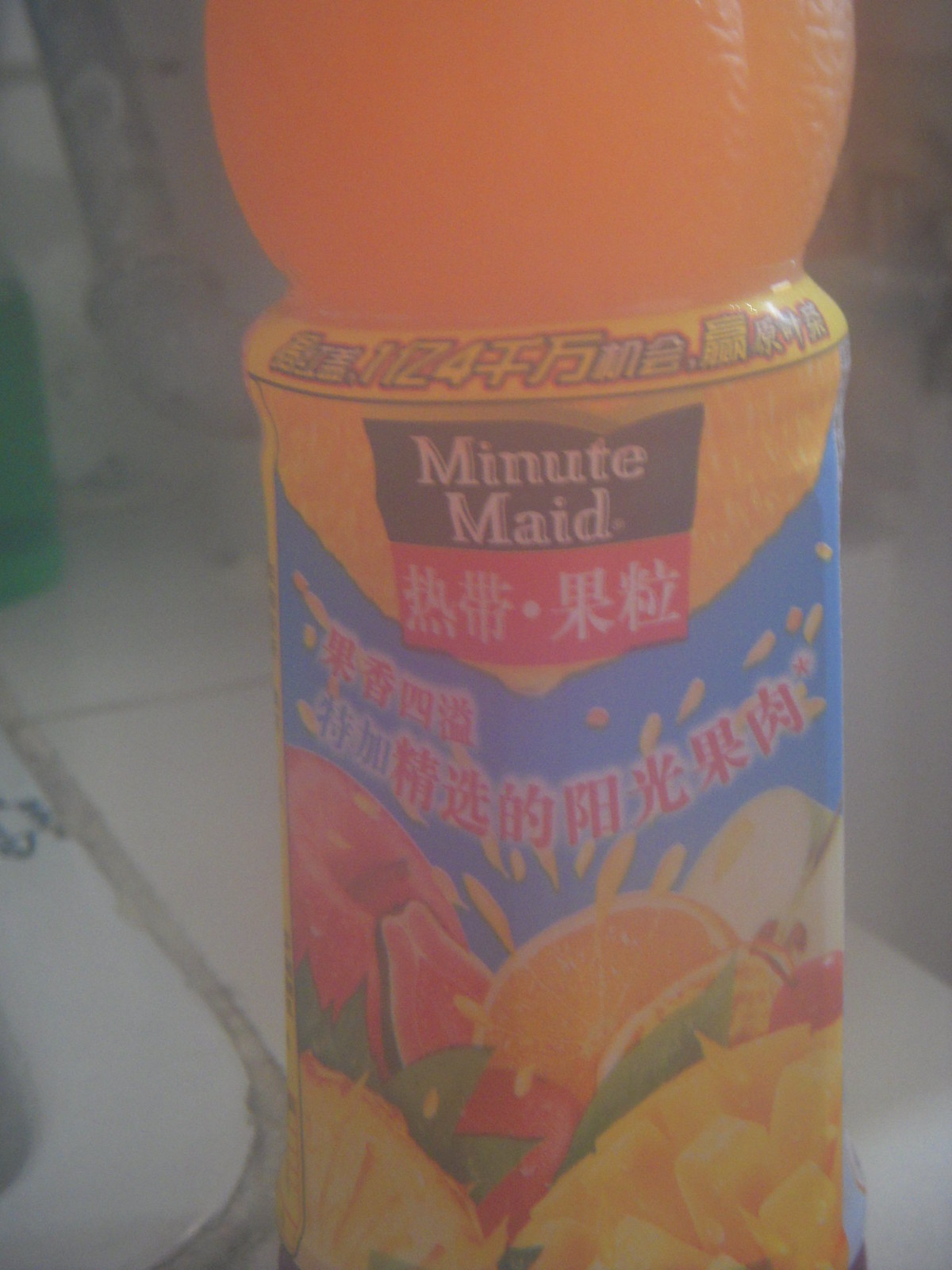The image features a Minute Maid drink prominently displayed against a somewhat dark background, which seems to vary in color from gray on the left to black on the right. The drink is set on a white tiled surface with distinct gray grout, possibly a table or countertop. The bottle is clear, containing a vibrant orange liquid, and crowned with a large, textured plastic orange resembling a globe. The front label of the bottle is colorful with a predominantly blue background. At the top, there is a black rectangular banner displaying "Minute Maid" in white text. Below that, red Asian characters are inscribed, likely Chinese, within a triangular blue banner. The lower portion of the label features images of various fruits including oranges, a pineapple or possibly dragon fruit, strawberries, and what might be a guava, with yellow droplets indicating their juiciness. The label also contains additional Asian script outlined in black, highlighting the drink's multicultural branding.